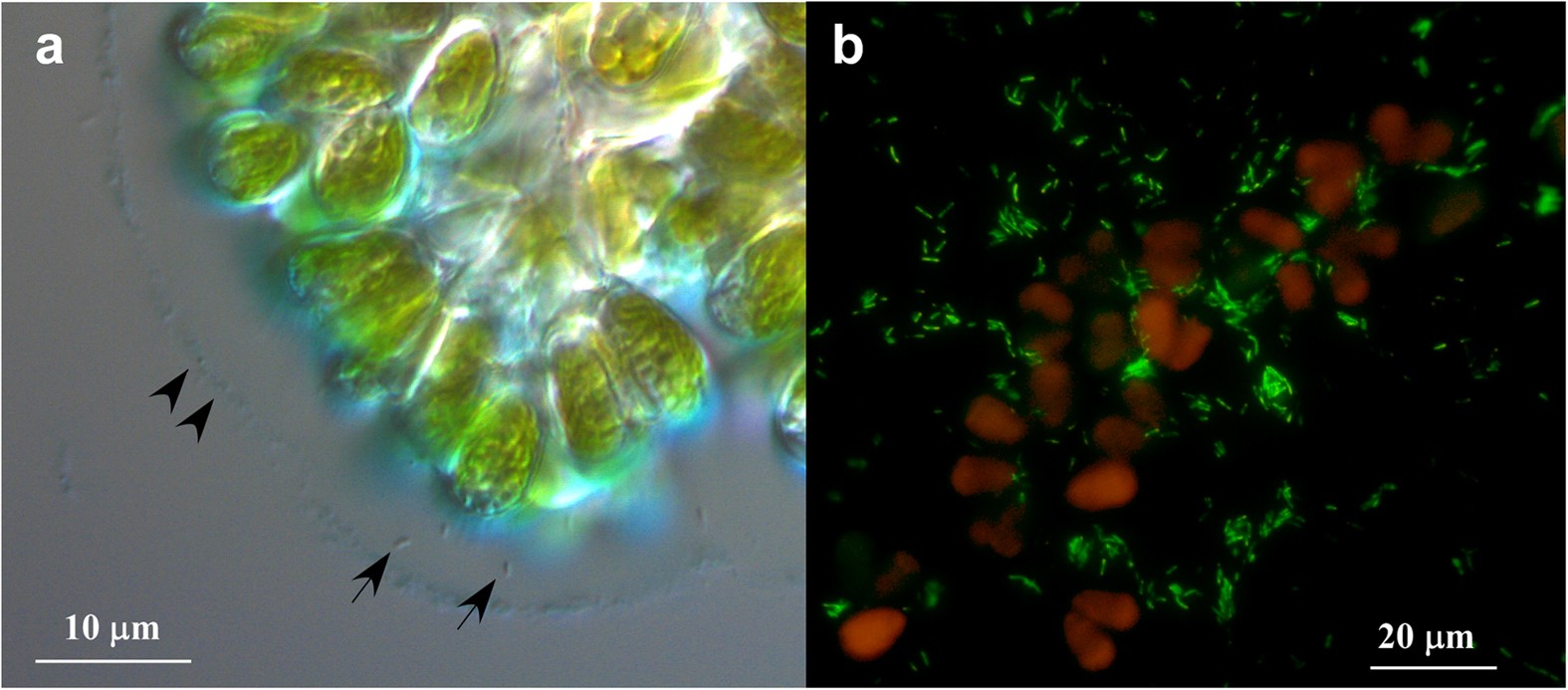The composite image consists of two side-by-side micrographs labeled 'A' and 'B'. In micrograph A, the label 'A' is positioned in the upper left-hand corner in white. The scale bar on the bottom left indicates a measurement of 10 micrometers. This image reveals a light-colored surface populated by numerous green circles and ovals, each outlined in white. Four arrows are visibly pointing to specific points of interest within this microscopic landscape.

Micrograph B, labeled 'B' in the upper left-hand corner with a white 'B' and featuring a scale bar indicating 20 micrometers, exhibits a stark contrast. The background is predominantly black, giving the impression of a dark, neon-lit scene. Within this dark backdrop, green areas are interspersed with vibrant, neon orange specks, creating a striking display of color against the black surface.